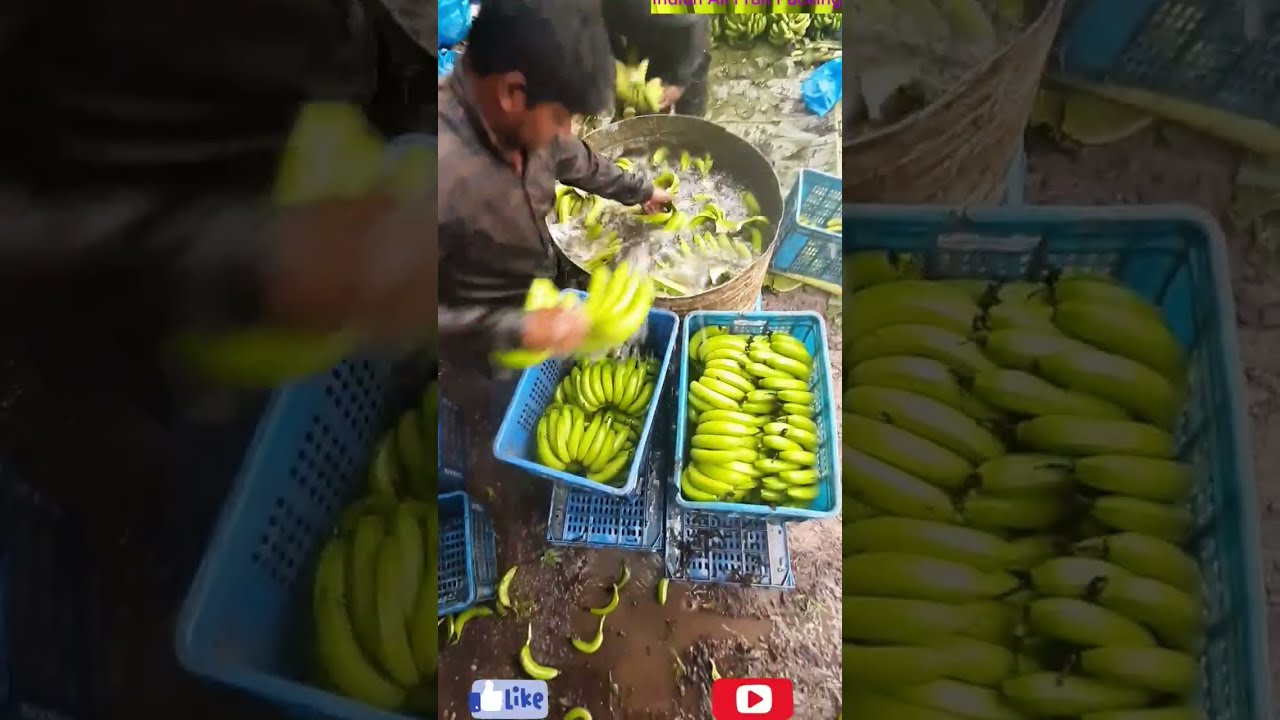In this outdoor image, a man with very dark hair and a dark shirt, possibly Indian, is seen washing bananas. He stands at the top-left of the frame, focused on his task amidst a muddy ground with puddles and scattered bananas. The man uses his left hand to immerse bananas into a large steel barrel filled with water, while his right hand holds another bunch of bananas, seemingly in motion as the photo was taken. Two blue plastic crates filled with bushels of bananas are placed nearby, possibly to his right, indicating a diligent process of cleaning and sorting the fruit. In the background, the torso, thigh, and hand of another person engaged in the same activity are faintly visible. The bottom of the image features a Facebook-like icon on the left and a YouTube play button on the right, both accompanied by a blurred, wide border on either side that appears to be an enlarged and out-of-focus extension of the main image.